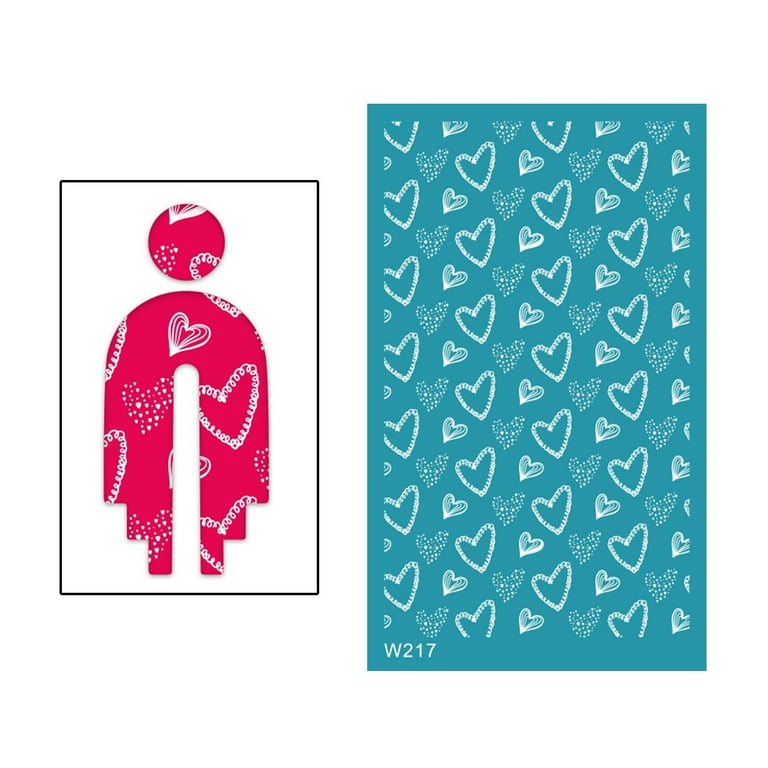The image is composed of two distinct sections, each featuring unique shapes and designs. On the left side, a black rectangle stands tall with a predominantly white background. Within this rectangle, at the top, is a pink circle adorned with white hearts formed by squiggly lines and dots. Below it, there's an upside-down horseshoe or an inverted 'U' shape in pink, which also features white hearts with similar squiggly lines. The bottom of this inverted 'U' has stair-like structures leading towards the center. On the right side, the entire background is a teal blue, filled with white hearts crafted from squiggly lines and dots. Additionally, the bottom left corner of this teal rectangle has the text "W217" written in white. This composite image skillfully combines contrasting colors and intricate heart patterns within geometrically distinct shapes.